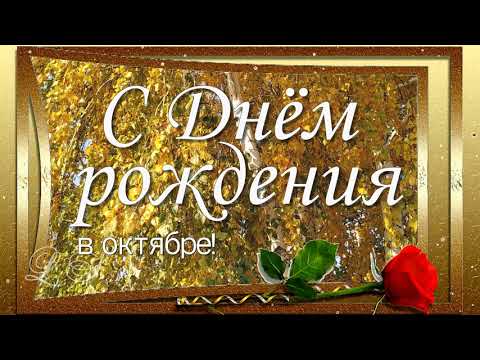This image displays an intricately designed piece of framed artwork. The artwork features a peculiar double-framed structure: the outer frame is a simple rectangle, while the inner frame has an artistically warped design with the left edge, top, and bottom all curving inward, the right edge remaining straight. The inner frame encloses a background that is a striking gold gradient combined with autumn leaves in various yellow and gold shades. Superimposed on this backdrop is large Russian text, splitting into two lines and offering an enigmatic message written in reversed and capitalized characters. Adding to the complexity, a red rose with a green stem and three green leaves lies horizontally at the bottom of the outer frame, adorned with a gold ribbon wrapped in a serpentine manner, and a corkscrew emerging from its end. The entire composition blends elements of abstract art and elaborate graphic design, creating a visually engaging and thought-provoking image.